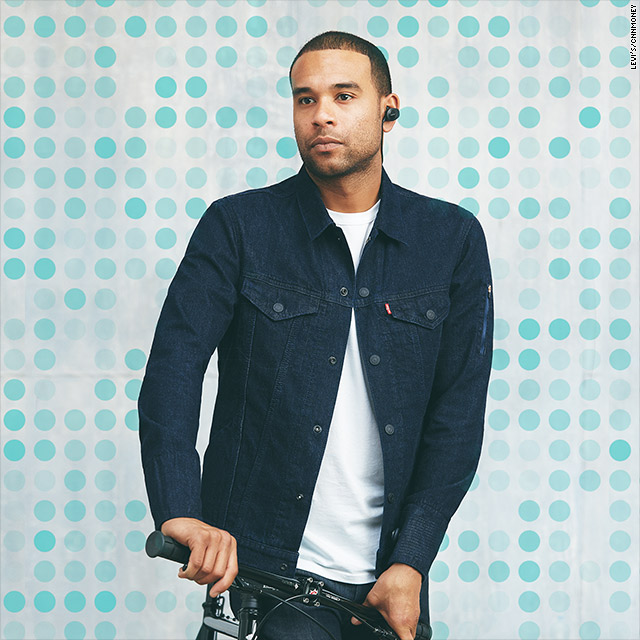This detailed image features a man with medium tan skin, short cropped black hair, and small black earbuds in his ears. He is dressed in a white t-shirt underneath an unbuttoned dark blue denim Levi's jacket, which prominently displays the red and white Levi's label on the left chest pocket. The man is holding the handlebars of a bicycle, although only the top of the bicycle, including the handlebars and the partially obscured seat, is visible. His hands rest on the handlebars, suggesting a casual lean or seated position to the right side of the bicycle. His black pants complete his outfit. 

The man, who could be mistaken for an actor or model due to his composed demeanor and attire, is gazing off into the distance with his mouth closed and his brown eyes directed slightly to his left. The background of the image is characterized by a polka dot pattern composed of alternating light green, dark green, and teal dots, some of which are faded, giving them a grayish appearance. This backdrop forms a harmonious contrast with the man's attire and adds a playful yet structured element to the overall composition.